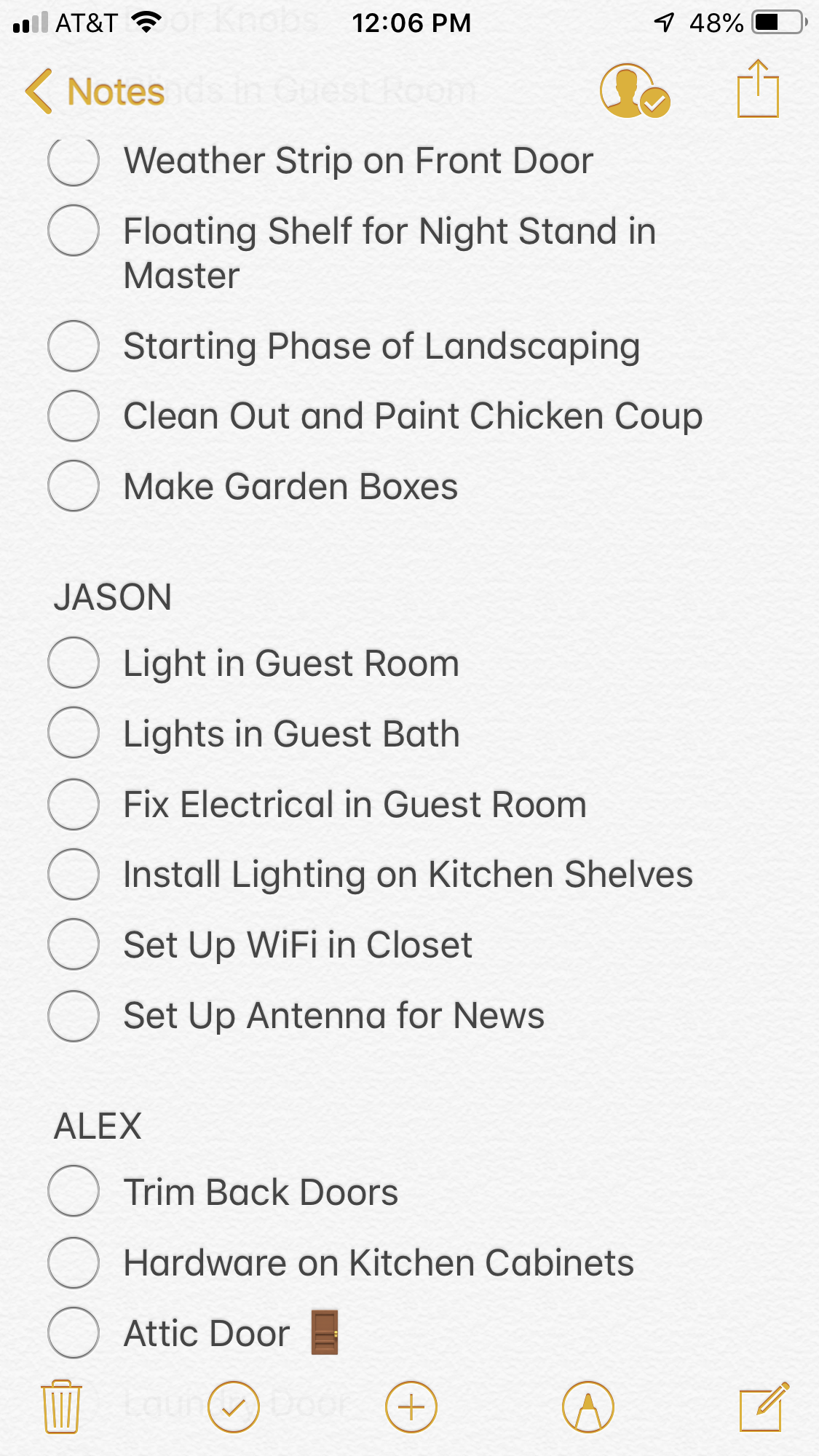**Caption:**

An iPhone screenshot displaying the "Notes" app is shown. The top status bar reveals the device's connectivity and battery information: the carrier is AT&T with two bars of cell service, full Wi-Fi signal, and the time is 12:06 PM. On the far right, an icon indicating tracking or navigation is active, and the battery percentage is at 48%.

Below the status bar, the interface of the Notes app is visible. The header in yellow displays the word "Notes," flanked by several icons: a back arrow on the left, followed by a person icon, a check mark inside a yellow circle, and an upload or share icon.

In the main body of the note, several to-do items are listed with bullet points under different sections:

- **First Section:**
  - Weatherstrip on front door
  - Floating shelf for nightstand in master
  - Starting phase of landscaping
  - Clean out and paint chicken coop
  - Make garden boxes

- **Second Section - Jason:**
  - Light in guest room
  - Lights in guest path
  - Fix electrical in guest room
  - Install lighting on kitchen shelves
  - Set up Wi-Fi in closet
  - Set up antenna for news

- **Third Section - Alex:**
  - Trim back doors
  - Hardware on kitchen cabinets
  - Attic door (accompanied by a digital image of an attic door)

At the bottom of the screen, various feature icons for the Notes app are displayed, including a trash can, a circle with a check mark, a circle with a plus, a circle with a pen tip, and a writing icon.